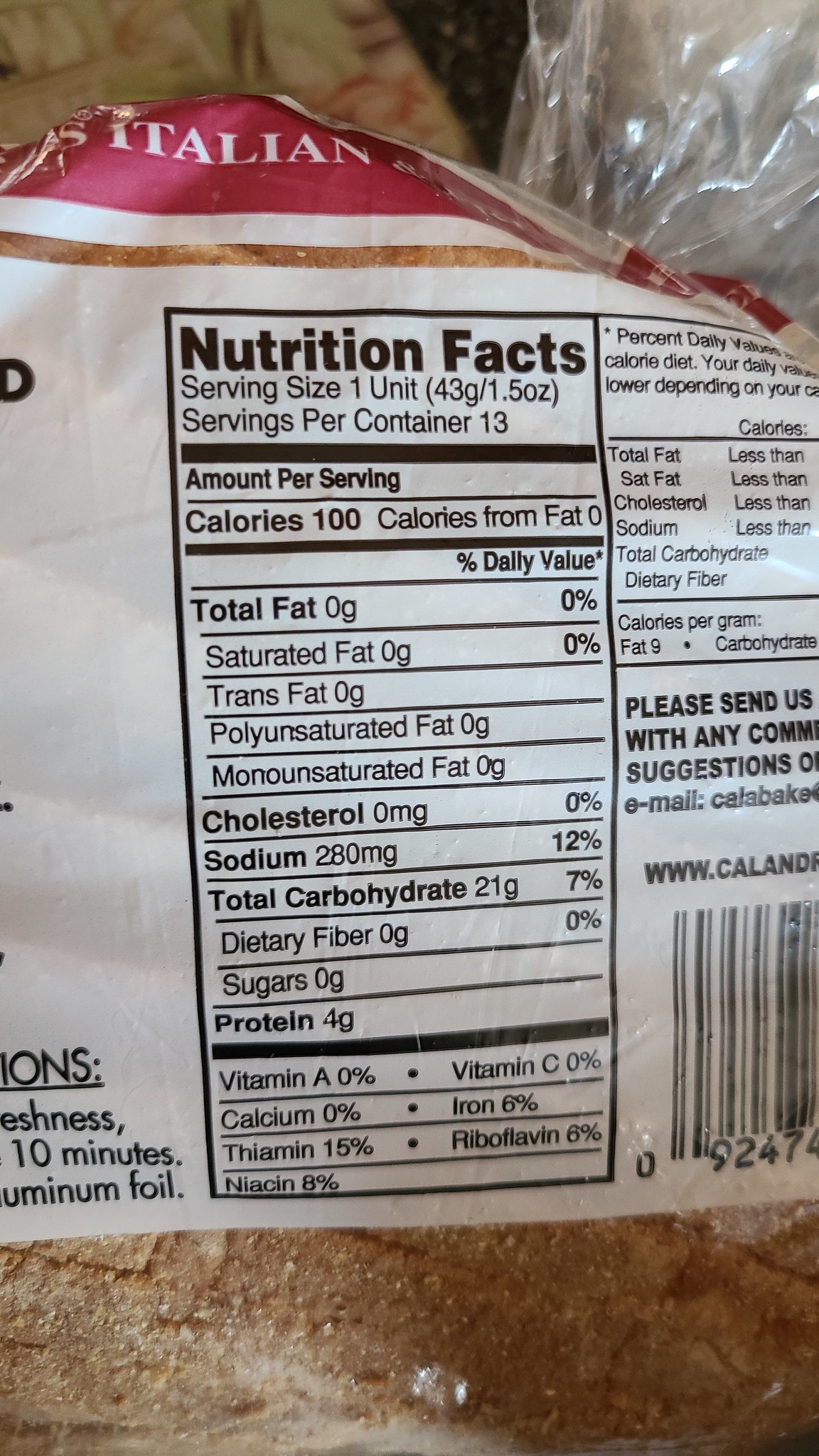The image is a vertically rectangular frame showcasing a clear plastic bag containing a loaf of bread. The loaf inside is a beautiful golden brown, exuding a freshly baked appearance typical of premium bread. The plastic bag is primarily transparent, making the loaf's inviting color and texture clearly visible. At the bottom portion of the frame, just above the loaf, is a white label which prominently displays the Nutrition Facts box. Further up, there is another segment of the clear plastic allowing an uninterrupted view of the bread's upper portion. Above this clear section, a thin white strip separates the view of the bread from the branding area. The topmost part of the bag features a red band with the word "Italian" printed in white lettering, underscoring the loaf's variety. The meticulous packaging not only protects the bread but allows an enticing preview of its delicious contents.